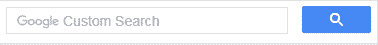The image depicts a section of a web page primarily consisting of a gray text box labeled "Google Custom Search." The familiar Google logo appears within this text box but rendered in gray rather than its usual colorful palette. The search box itself features a blue background with a white magnifying glass icon, indicating its purpose as a search field. Surrounding this search box is a border adorned with a pattern of small black and gray dots, which forms a distinct line around the box. Positioned above the dotted border is a more solid line, rendering the entire search box as a wide, rectangular shape. The overall page rests on a clean, white background typical of a website or computer interface. Adding to the layout, the image is framed by a gray-colored border, seamlessly blending with the gray and white text elements. The only significant color contrast within the image is the blue background of the search area, which prominently features the white search icon. This composition suggests functionality, allowing for text input in the search field.